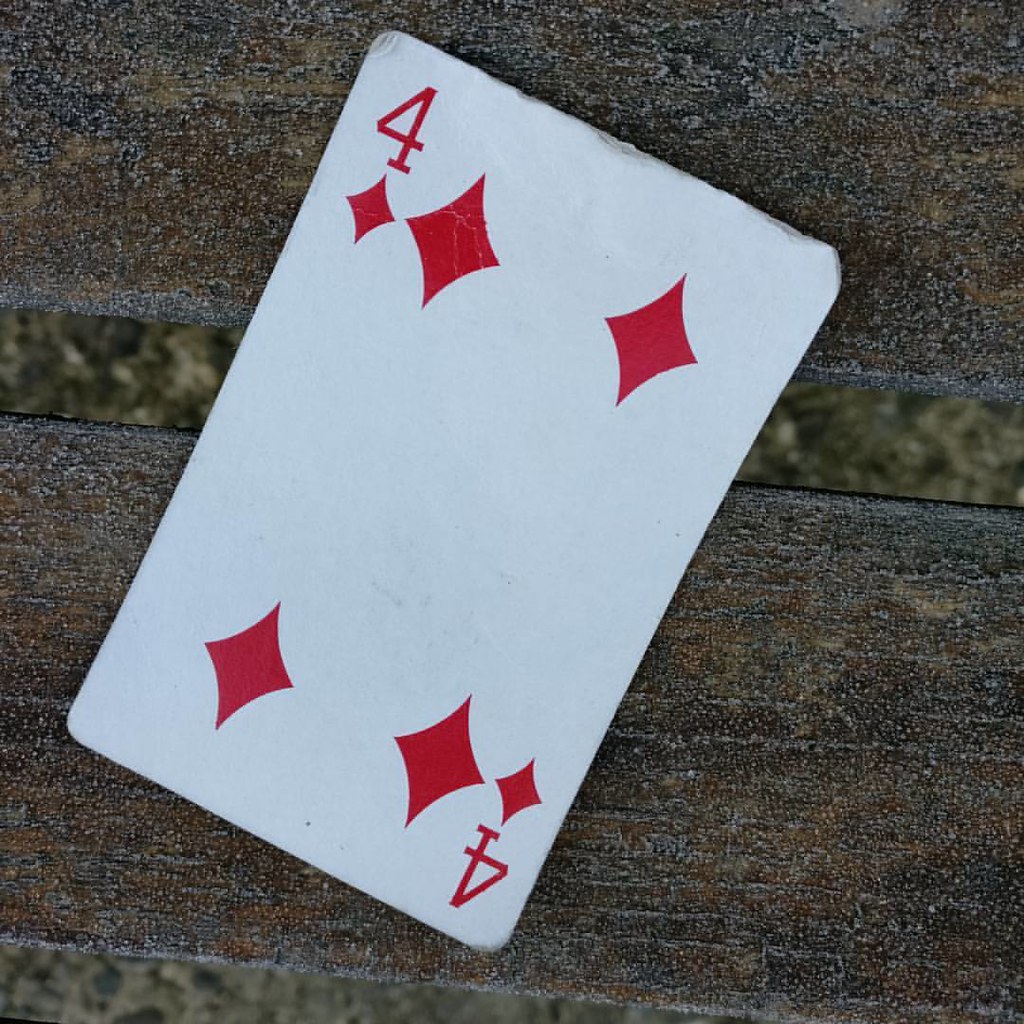A well-worn four of diamonds playing card is prominently displayed on a dark wooden surface, which has an olive green tinge to its brown color. The card, positioned diagonally with its upper left and lower right corners touching the top and bottom of the frame, respectively, shows signs of use. A closer look at the upper left diamond reveals subtle cracking in the print, and the entire upper edge of the card appears rounded and worn, suggesting frequent handling. In contrast, the rest of the card remains in pristine condition. The table, possibly aged, features metal straps running horizontally across the image, possibly indicating joints or reinforcements between the wooden boards. These metal strips have a pronounced greenish tint, adding to the rustic character of the scene. There are at least two of these bands visible, with one located toward the lower part of the image. The overall composition is simple yet sharply focused, highlighting the textures and details of both the card and the wooden surface.